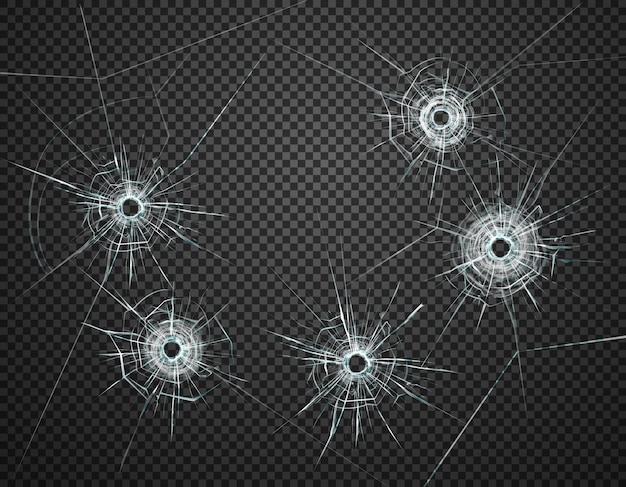This digitally enhanced rectangular photograph presents a striking three-dimensional view akin to peering through a clear glass windshield that has been shot five times in a circular formation. The shattered bullet holes create a dramatic foreground, with intricate spiderweb-like cracks radiating from each point of impact. Beyond the fractured glass lies an array of meticulously detailed black and gray checkerboard patterns. The checkerboard squares are exceptionally small and finely lined, so much so that approximately four tiny squares can fit within the diameter of a single bullet hole. In total, the image features well over a thousand of these minuscule squares, contributing to a visually compelling and complex composition.